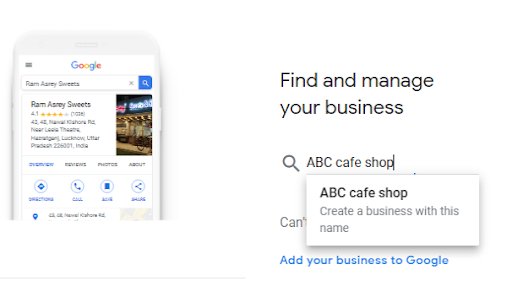The image displays the Google search results for "RAM ASNE Suites" (spelled R-A-M A-S-N-E-Y S-W-E-E-T-S). The establishment boasts a 4.1-star rating based on 1,026 reviews. The address appears to be 43, 42 Natural Clayhons Road near Lessee Theater, although the text is somewhat blurry and hard to decipher. The location is in Muzzleburg, Luckintown, with a postal code of 226001, India.

A photo of the business is prominently shown. Several interactive buttons are visible, including "Overview," "Reviews," "Photos," and "About." Additional buttons for "Directions," "Call," another unreadable option, and "Share" are also present.

On the right side of the image, there is a section titled "Find and manage your business," featuring a magnifying glass icon and repeated entries for "ABC Cafe Shop," suggesting the creation of a business listing with that name. Beneath this is a prompt encouraging users to "Add your business to Google."